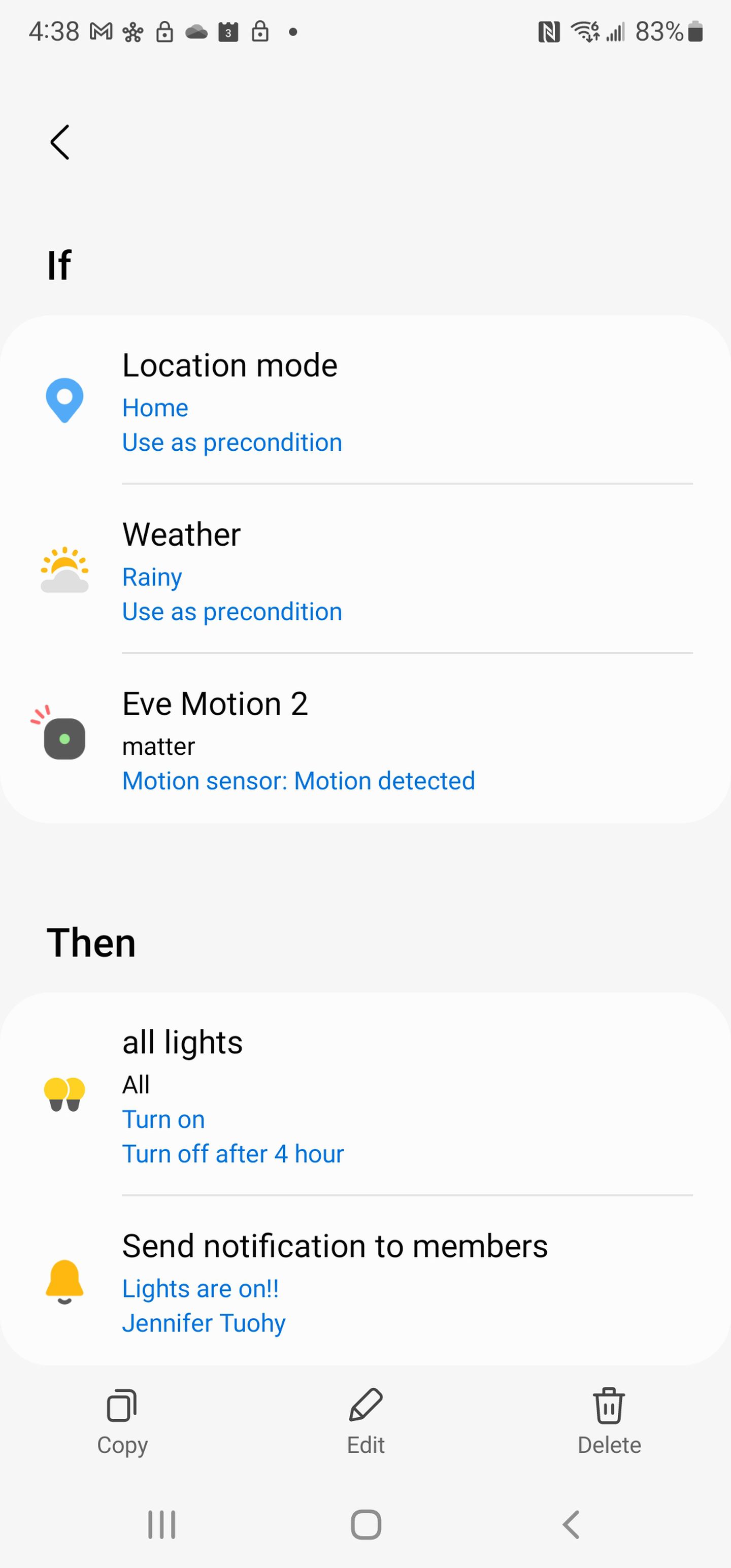This detailed screenshot showcases the interface of a smartphone application, most likely intended for managing smart home devices based on certain conditions. At the top left corner, the status bar displays the time, 4:38, along with various app icons. The battery indication on the right-hand corner shows 83% remaining. 

Below the status bar, a back-arrow icon is present for navigation. The display is divided into sections labeled "IF" and "THEN," facilitating conditional triggers for smart home automation. The "IF" section contains three tabs:

1. **Location Mode: Home** - Utilized as a precondition.
2. **Weather: Rainy** - Utilized as a precondition.
3. **Motion Detected** - From a motion sensor labeled "Eat Motion to Matter."

In the "THEN" section, the interface specifies actions to be taken when the conditions are met:

1. **All Lights** - This tab indicates that all lights will turn on and then turn off after four hours.
2. **Send Notification to Members** - Specifies that a notification will be sent to members, stating "Lights are on, Jennifer Tui."

Beneath these actionable sections are three buttons labeled: 

1. **Copy**
2. **Edit**
3. **Delete** (indicated with a trash can icon)

Further below, additional icons are present, seemingly part of the app’s interface. These include three horizontal lines, a square with rounded corners, and a left-pointing arrow, each likely representing different functions or navigational tools within the app.